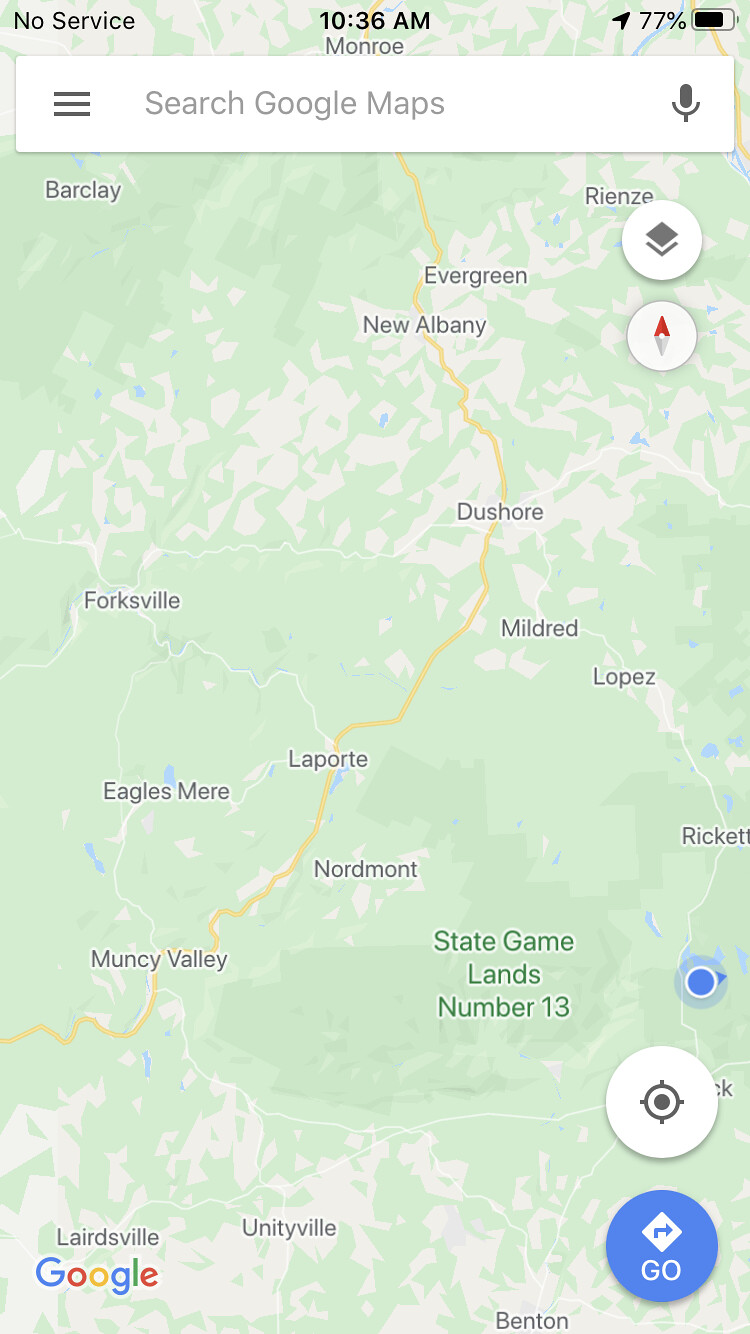The image appears to be a screenshot from a GPS navigation app, likely from Google Maps. It displays a map with various town names such as New Albany, Evergreen, Deshmore, Folksville, Mildred, Lopez, and Laporte. The map is styled in vector graphics, showcasing multiple shades of green to distinguish different terrains or areas. The roads are depicted in a gold color with a black border, making them easily identifiable. In the upper left corner of the image, the text "No service" indicates a lack of cellular network connectivity. The time is displayed as 10:36 a.m. In the upper right corner, a delta symbol represents the current location, accompanied by a battery icon showing 77% battery life remaining.